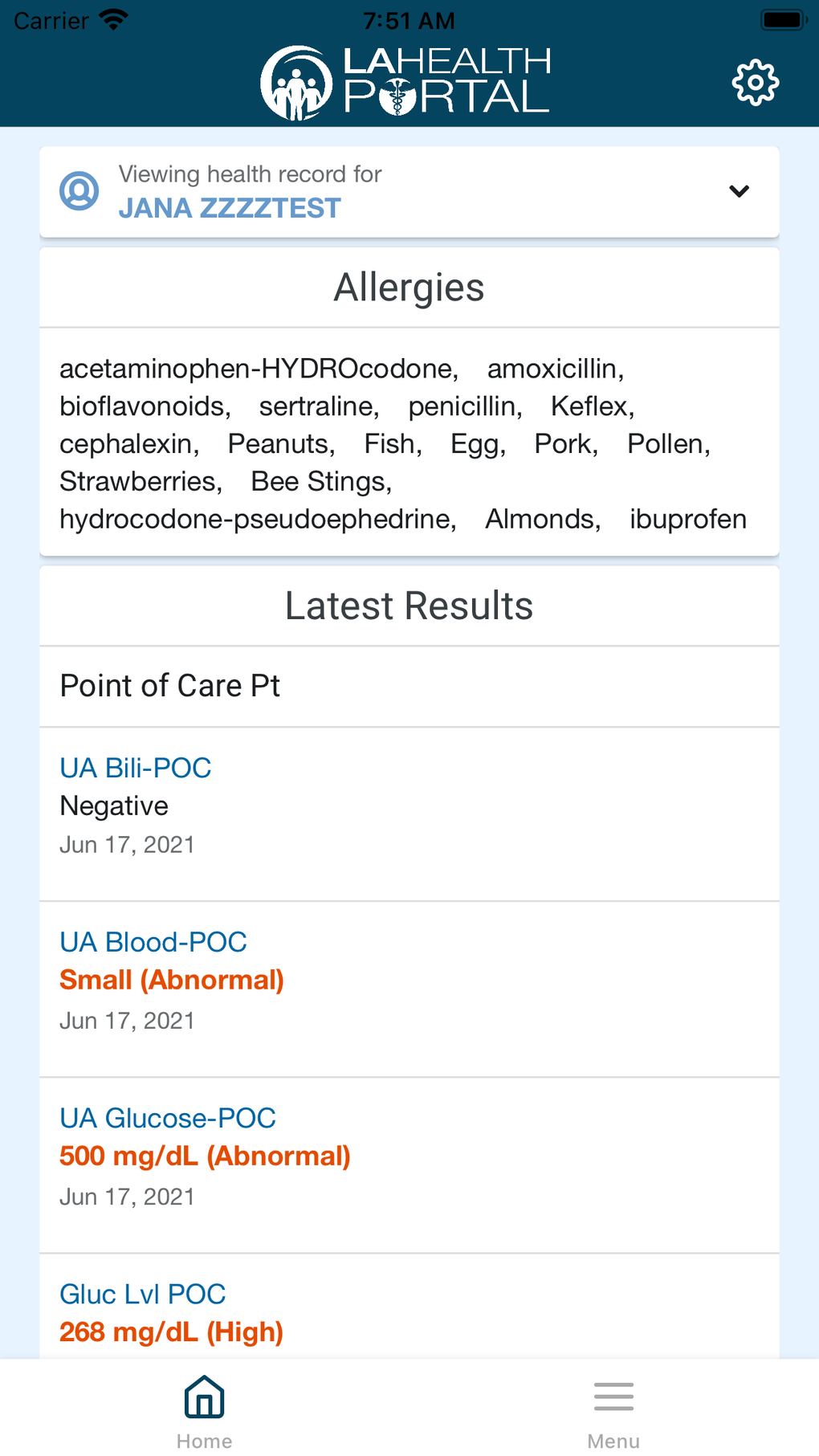This is a detailed screenshot from a cell phone display. The image is vertically elongated, approximately three times taller than it is wide. 

At the very top, a dark blue bar spans across the screen. In the upper left corner, the word "carrier" is displayed in black. Adjacent to it, the Wi-Fi signal icon appears in black. Centrally positioned, the time reads "7:51 AM" in black numerals. On the far right is the battery icon.

Below the time, "LA Health" is written, accompanied by a logo to its left, which depicts a circle with an outline of an adult in the center flanked by children. To the right of "LA Health," a white settings icon is visible.

The screen below features a light blue border along the top and sides. Inside this border, a white rectangle houses a blue circle with a person icon. Next to this icon, the text "Viewing Health Record" is displayed in black.

Following this, in bold, blue, all-capital letters, "JANNA ZZZ TEST" is prominently shown. Underneath, there's another square labeled "Allergies," listing five lines of allergies.

A small blue bar separates this section from the "Latest Results" area. Here, on the left side, it says "Latest Results" in white letters, while the right side reads "Point of Care" in black. 

Subsequent lines provide detailed health results starting with "UA BIL - POC," noted as "Negative," followed by the date. Each result is separated by thin gray lines:
- "UA Blood - POC": Marked in orange as "Small Abnormal," followed by the date.
- "UA Glucose - POC": Displayed with "500 mg/DL" in orange, noted as "Abnormal," followed by the date.
- "GLU C LVL - POC": Listed with "268 mg/DL" in orange, marked as "High," followed by the date.

Finally, at the very bottom, a white border contains two icons: a home icon on the left and a menu icon on the right.